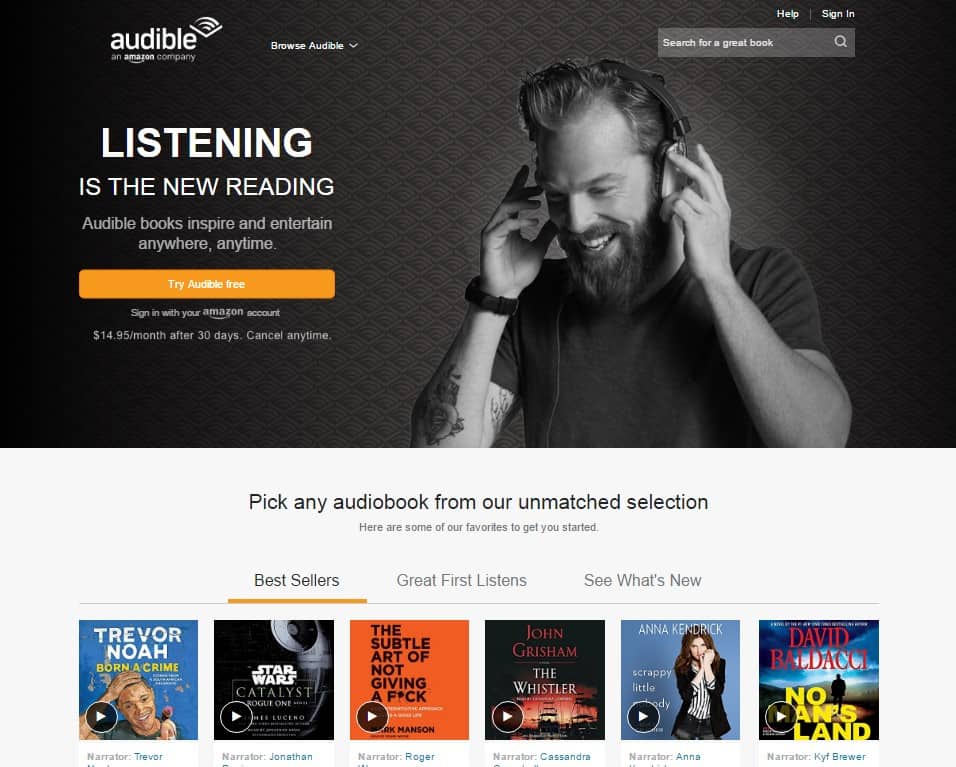The image depicts a detailed view of the Audible website, framed in a horizontal rectangular shape. The background features a dark charcoal gray hue which lightens slightly towards the center, exhibiting a subtle diamond pattern with 3D-like lines within the shapes.

In the top left corner, the white text "Audible" is displayed alongside the Audible logo, depicting an open book with soundwave lines emanating from it. Notably, it is indicated that Audible is an Amazon company. Moving rightward, the phrase "Browse Audible" accompanies a drop-down menu button. Further to the right, a search bar is located, with "Help" and "Sign In" options listed above it.

Beneath the search bar, an image of a smiling Caucasian man dominates the scene. Portrayed mostly from the front but slightly angled to show more of his left profile, he sports a beard and headphones while holding them with his hands. He is dressed in a t-shirt and wears a watch on his right wrist, the entire image rendered in black and white.

To the left of the man's image, bold text reads "Listening is the new reading. Audible books inspire and entertain anywhere, anytime." Below, a prominent orange button invites users to "Try Audible Free." Attached to this call-to-action, there's additional text indicating users can sign in with their Amazon account, noting the service costs $14.95 per month after a 30-day free trial, with the option to cancel anytime.

The surrounding light gray background communicates, "Pick any audiobook from an unmatched selection. Here are some of our favorites to get you started." Just below, there are tabs categorizing "Bestsellers," "Great First Listens," and "See What's New." Following these tabs, six suggested audiobooks are highlighted, showcasing Audible’s curated recommendations for listeners.